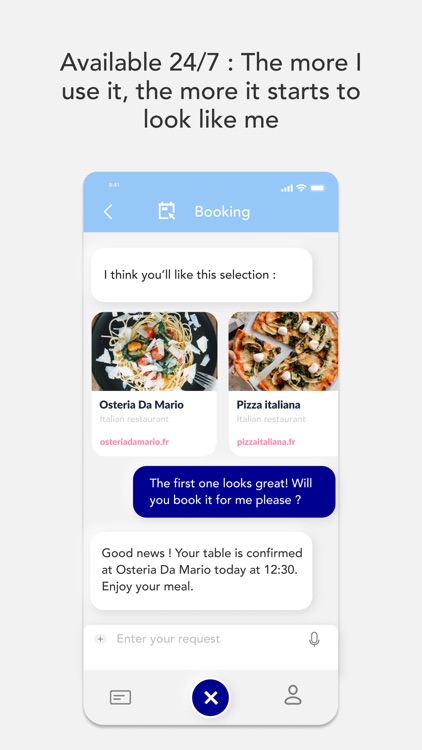In the image, a vibrant background frames a central feature, drawing the eye to the top-center text that reads, "Available 24-7." Below this, a screenshot captures a cell phone interface. The phone's status bar shows the time as 9:43 AM, with full cell signal, Wi-Fi strength, and battery life displayed in white icons. 

The main focus within the phone interface includes an arrow pointing left, leading to a calendar icon labeled "Booking." On a gray backdrop inside the phone, a white text box with black text states, "I think you’ll like this selection."

Beneath the text box are two food images: one of a pasta dish labeled "Orzata Di Mario," identified as an Italian restaurant in gray text with a blue hyperlink, and another of a pizza with a slice being taken out, labeled "Pizza Italiana," also underlined by "Italian restaurant" in gray and a blue hyperlink.

To the right of these images, another blue background features white text stating, "This one looks great. Will you book it for me, please?" Additionally, white text on the left side confirms, "Good news, your table is confirmed for Orzata Di Mario today at 12:30. Enjoy your meal."

The bottom of the screenshot includes a gray box for typing requests and a gray microphone icon. Beneath this, a conversation bar displays a blue circle with a white X and a silhouette icon on the right side.